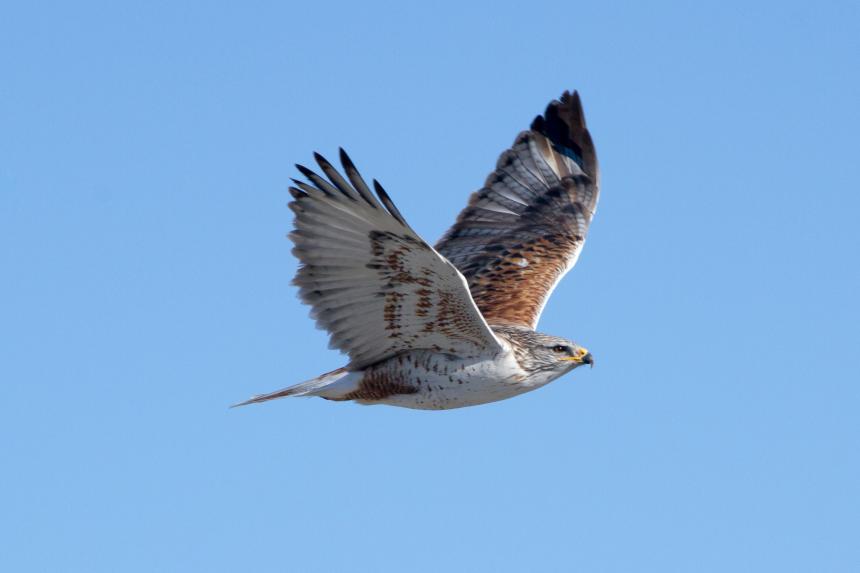This image captures a bird in mid-flight against a clear, baby blue sky without a cloud in sight. The photograph is taken very close-up, allowing a detailed view of the bird’s side, including its sharp, curved beak and its right eye. The bird, possibly a hawk, falcon, or eagle, exhibits a graceful yet powerful presence with its wings fully extended. The wings display a fascinating mix of colors: the undersides are primarily white with speckled brown and black patterns, while the upper parts are brown towards the front feathers and grayish towards the back. The bird's body is mostly a cream or white color, speckled with brown, and its head carries a pattern of gray speckled with white. Sunlight bathes the bird, accentuating the intricate details and vibrant hues of its plumage, making it the sole focus against the vast expanse of the blue sky.